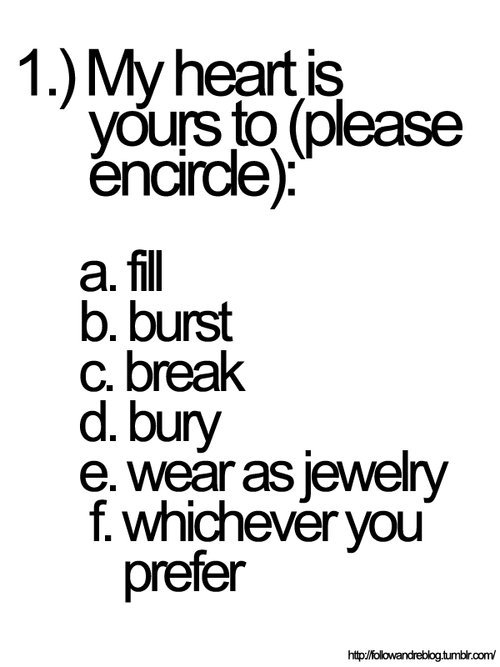The image is a simplistic internet meme featuring black text on a white background. At the top, it reads "1) My heart is yours to" followed by "please encircle:" in parentheses. Below are six multiple-choice options labeled A through F, each preceded by a period:

A. Fill  
B. Burst  
C. Break  
D. Bury  
E. Wear as jewelry  
F. Whichever you prefer

The intention of the meme is to complete the sentence by selecting one of the options. At the bottom, a web address is displayed: "http://followandrebecca.tumblr.com." This quirky multiple-choice meme has a straightforward design, likely shared on social media platforms as a lighthearted or thought-provoking post.